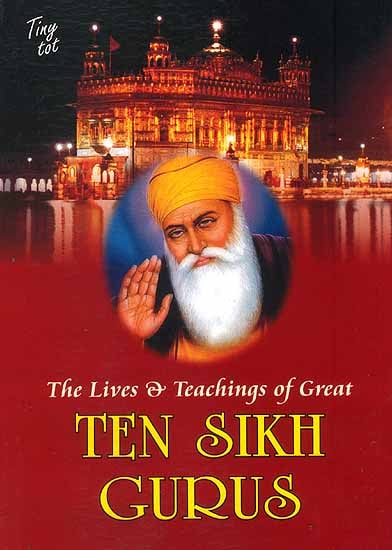The image is likely a book jacket cover featuring a harmonious blend of photography and illustration. At the top of the rectangular cover, set against a dark, night sky, the title "Tiny Tot" appears in elegant white script in the upper left corner. Below this, a majestic, ornate castle dominates the upper half of the cover. The castle, three stories high and well-lit, is dramatically framed by the dark sky with its lights reflecting off a body of water in the foreground, creating a captivating, luminescent effect.

Central to the cover, overlaid on the lower portion of the castle, is a circular illustration of a man waving and looking directly at the viewer. He has a large white beard and mustache, with blue eyes and a slightly darker skin tone. He is adorned in a gold-colored head wrap and a yellow shirt beneath a dark shawl or robe, giving him a distinguished appearance. The background of the circular illustration is a contrasting blue hue.

The bottom portion of the cover transitions to a striking red background. Displayed prominently in white font are the words "The Lives and Teachings of Great," followed by "Ten Sikh Gurus" in larger, bold yellow font.